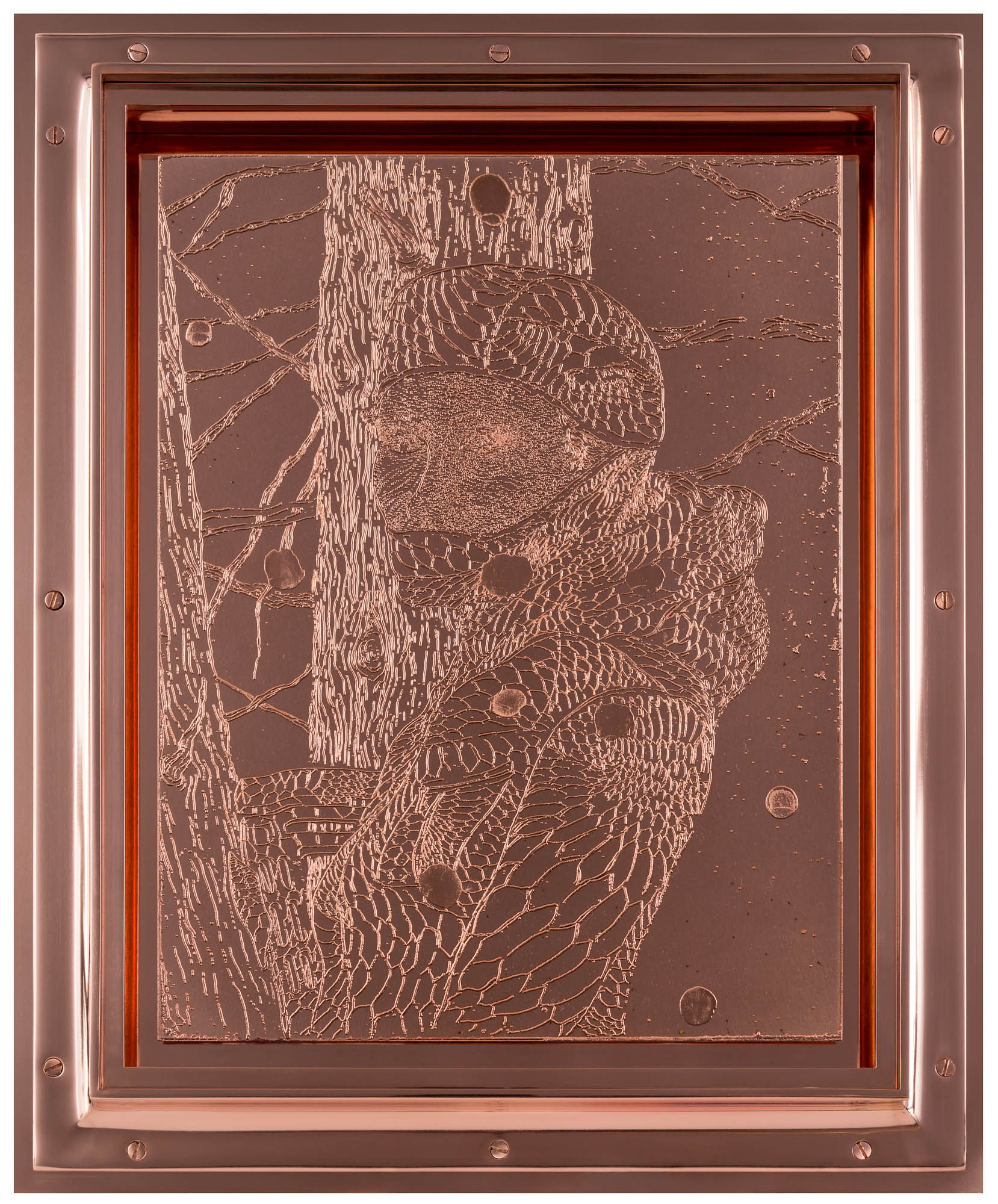The image features an intricately detailed metal etching, prominently framed in copper, with visible copper screws. Entitled "Diana, State 1" by Matthew Barney, created in 2018, this conceptual and figurative artwork captures a mysterious woman rendered on a monochrome copper plate. The central figure appears to merge both human and lizard-like features, dressed in robes resembling lizard skin. Her enigmatic gaze meets the viewer over her left shoulder, her face partly concealed by a mask and a scarf or cap. The complex texture of her outfit suggests cell-like elements, blending organic patterns with the metallic medium. Behind her, a tree trunk with branching limbs adds a natural contrast to the figure’s abstract form, extending from the top to the bottom of the image. The entire composition, set against a medium to dark copper backdrop, melds modern artistry with a sense of timeless mythology.